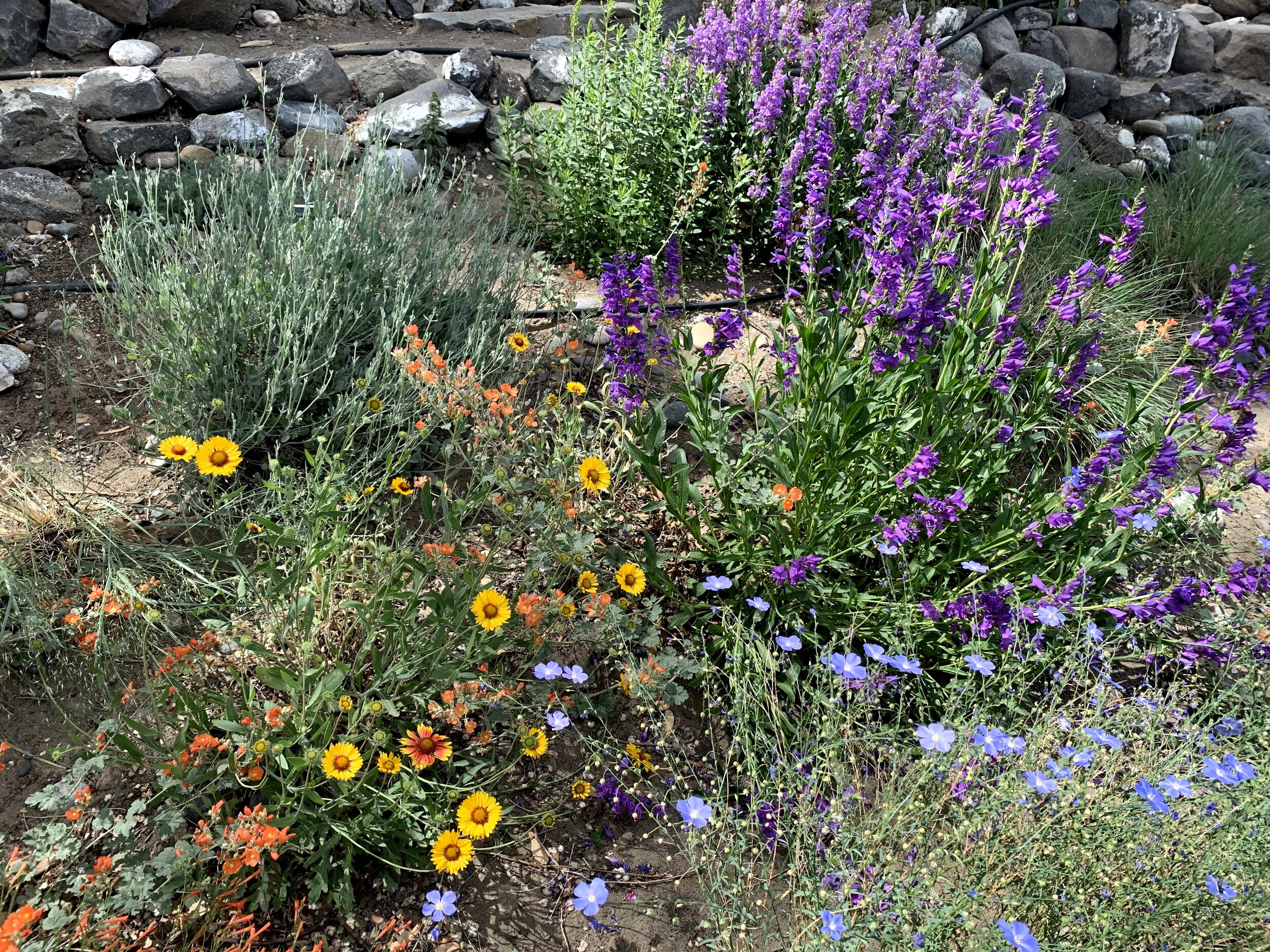This vibrant outdoor garden scene features a stunning array of flora against the backdrop of a meticulously constructed stone wall comprising large, grey rocks. The terrain around these rocks is a mixture of dirt and patches of sparsely grown grass, suggesting a natural setting. The garden, situated on a slight hill, boasts a variety of plants including bushes with bright purple flowers and clusters of light blue periwinkle blooms located in the bottom right corner. Scattered throughout are tall, well-cared-for plants bearing yellow flowers with orange centers, evocative of sunflowers, as well as some orange flowers that resemble their sunny counterparts. The green grass and stems weave through this colorful tableau, basking in the natural sunlight that highlights the stones on the left side of the image.